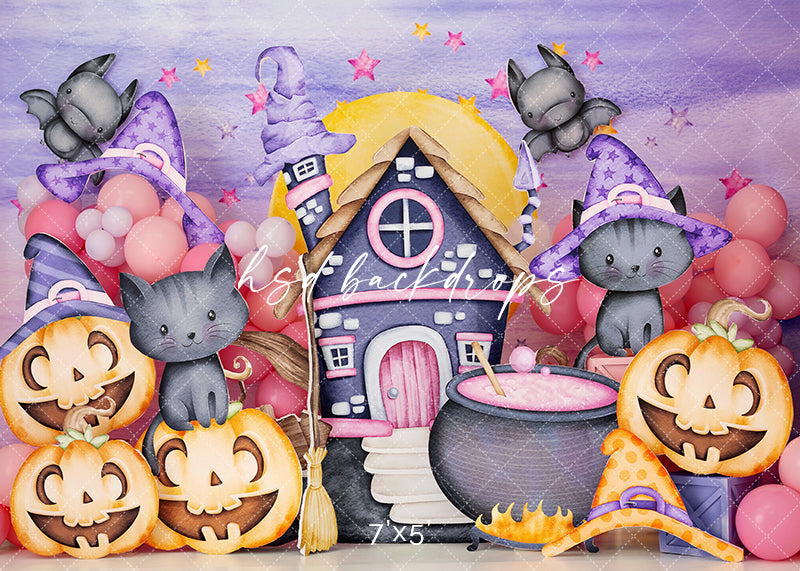The whimsical image features a brightly colored, cutesy cartoon scene with soft, pastel tones. At the center stands a charming black house accented with pink details, including a pink door, against a backdrop of a rising sun. Surrounding the house, a collection of smiley jack-o'-lanterns adds to the festive atmosphere. One of the pumpkins is topped with a purple witch hat adorned with light pink stars and a pink ribbon. Scattered throughout are small, grayish kittens, one of which is also wearing a similar purple witch hat.

A large cauldron, bubbling with pink liquid, sits prominently in the scene, contributing to the Halloween theme. Light-colored bats and whimsical stars in shades of pink, purple, and yellow dot the purple sky, enhancing the magical vibe. The top portion of the image features the text "HSD Backdrops" in white, while the bottom center portion indicates the dimensions "7x5." This playful arrangement, complete with bats, black cats, and witch hats of various colors and designs, evokes a delightful, spooky charm.